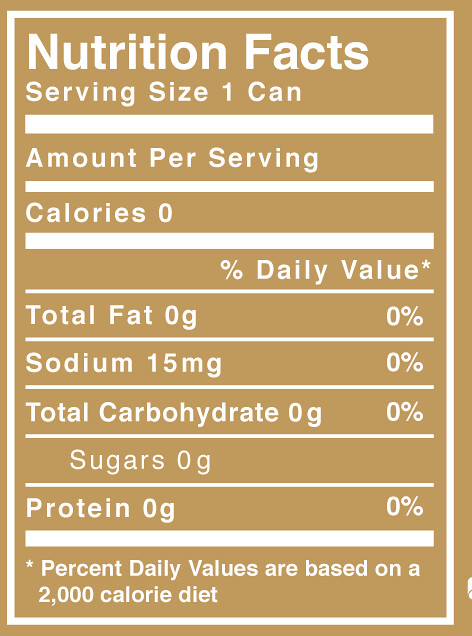This image shows a Nutrition Facts label on a mustard-beige or brown background with detailed white text and horizontal white bars dividing the information. The label starts with "Nutrition Facts" at the top, followed by "Serving size: one can." The "Amount per serving" section indicates zero calories, zero total fat, 15 milligrams of sodium, zero total carbohydrates, zero sugar, and zero protein. All values are separated by thin white horizontal bars. At the bottom, it states, "Percent daily values are based on a 2000 calorie diet." The edges of the label feature a narrow white rectangle border, with a tiny indentation visible at the lower right corner. The image is rectangular and possibly serves as a template, as it lacks specific product identification and most nutritional values are zero.